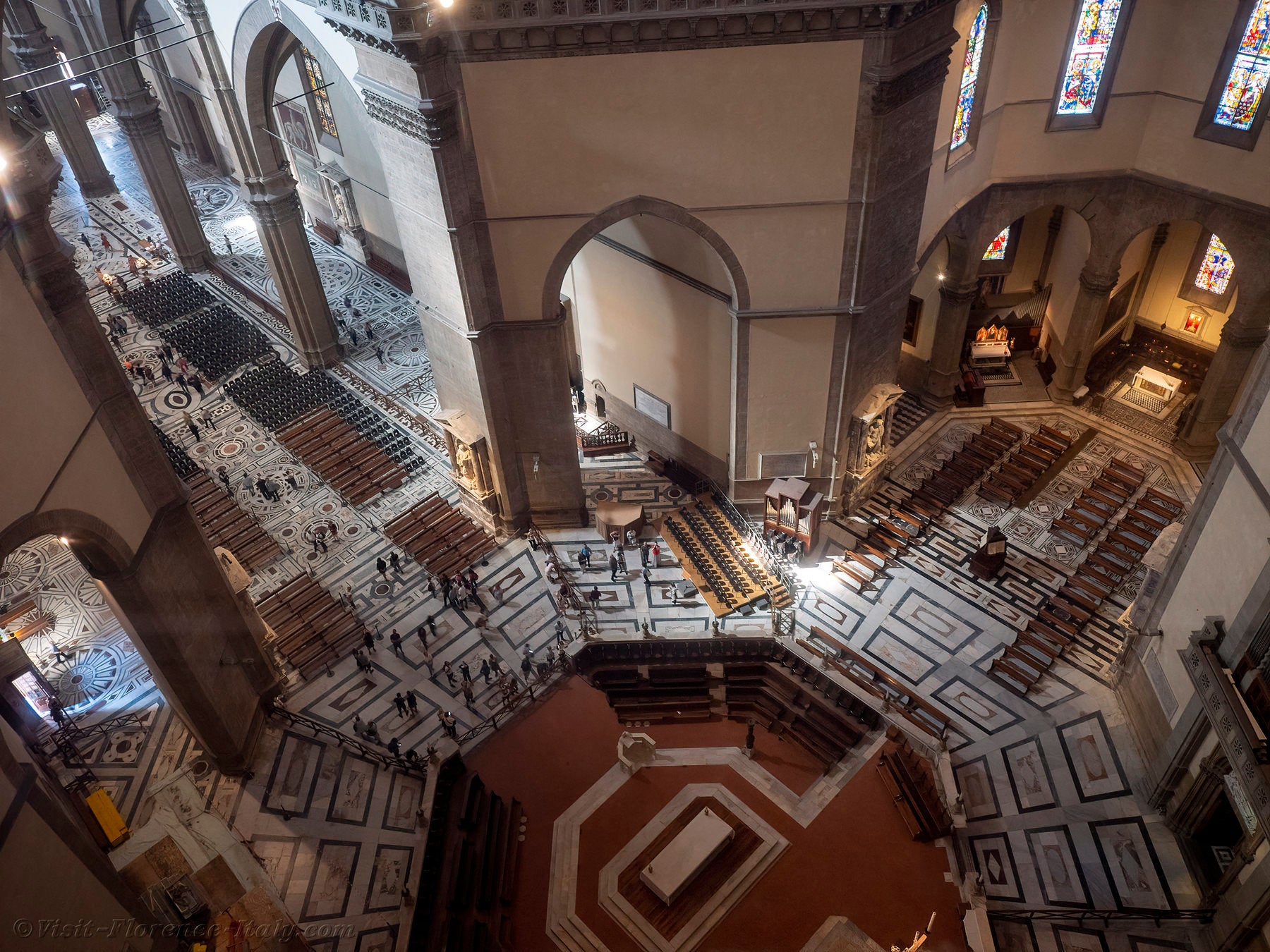This photograph captures the interior of a grand, ornate cathedral from a high, top-down perspective. The center of the image prominently features an octagonal altar area, adorned in varying shades of tan and dark brown, drawing the eye immediately to its intricate design. The expansive floor, patterned with delicate, detailed rectangles, leads the gaze to multiple areas within the cathedral. To the right, a sanctuary area with rows of pews is visible, and to the left, additional rows of pews merge with a section of neatly arranged chairs. Despite it not being a time for mass, some visitors can be seen scattered throughout, emphasizing the cathedral's attraction and significance. The building's age and preservation are evident, with majestic archways guiding people to different sections and beautiful stained glass windows adding to its historic charm.